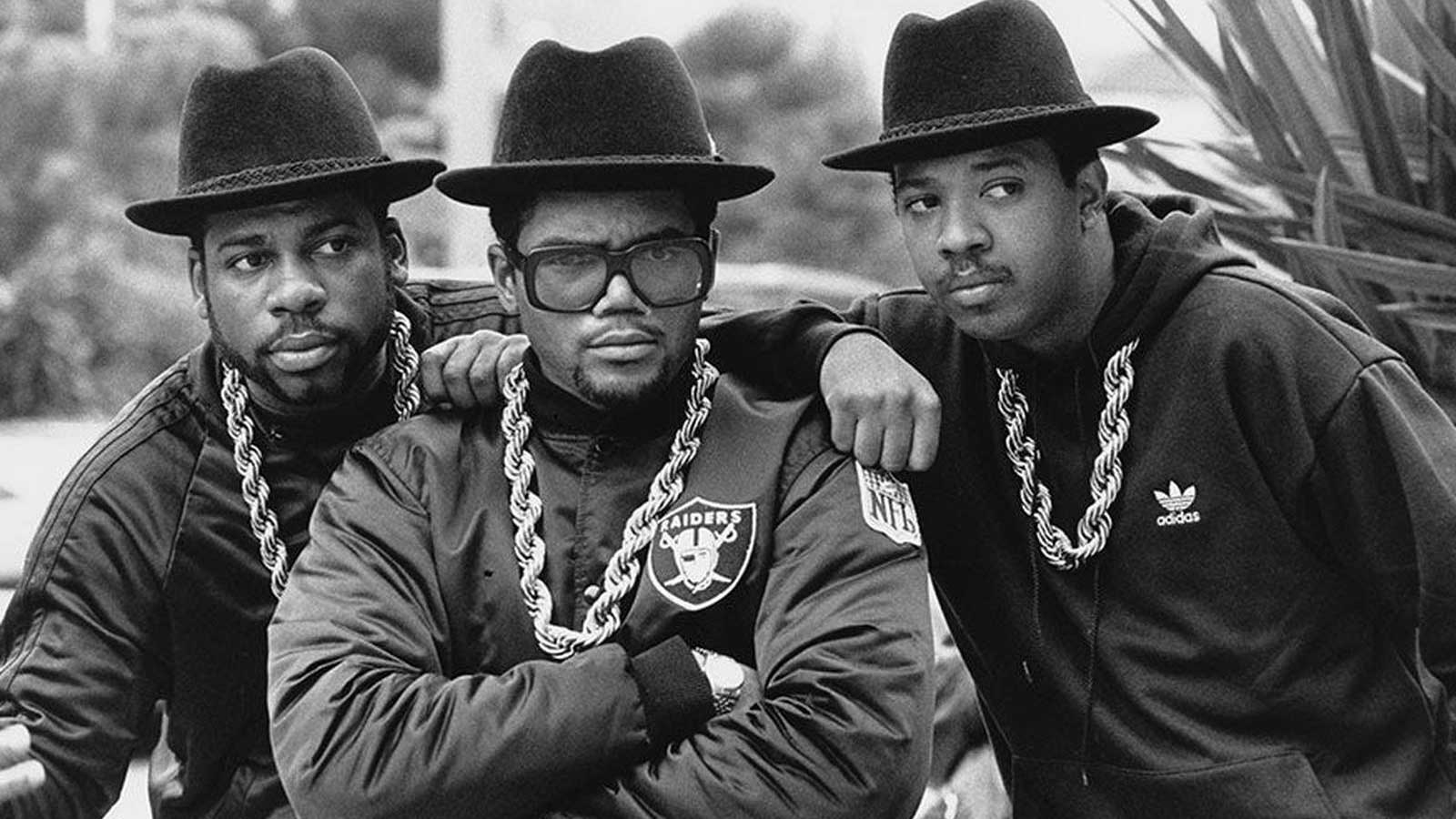This black-and-white photograph features the iconic hip-hop group Run-DMC. The image captures the three members standing together in front of a backdrop of out-of-focus foliage, including trees and possibly a palm tree. Each member is wearing their signature black hat and a large, thick gold chain around their necks. The man on the left has a thin beard and is dressed in a dark jacket with a hand resting on the shoulder of the man in the middle. He appears to be looking off to the right. The central figure commands attention with large black-framed glasses, a Raiders jacket, a giant chain, and a watch peeking out from his folded arms. His expression is intense, looking straight ahead. The man on the right, sporting a dark Adidas hooded sweatshirt and a faint mustache, also places his arm on the man in the middle’s shoulder and looks off to the right. The trio's poses and attire align with Run-DMC's iconic look, making this likely a promotional or album cover photograph.